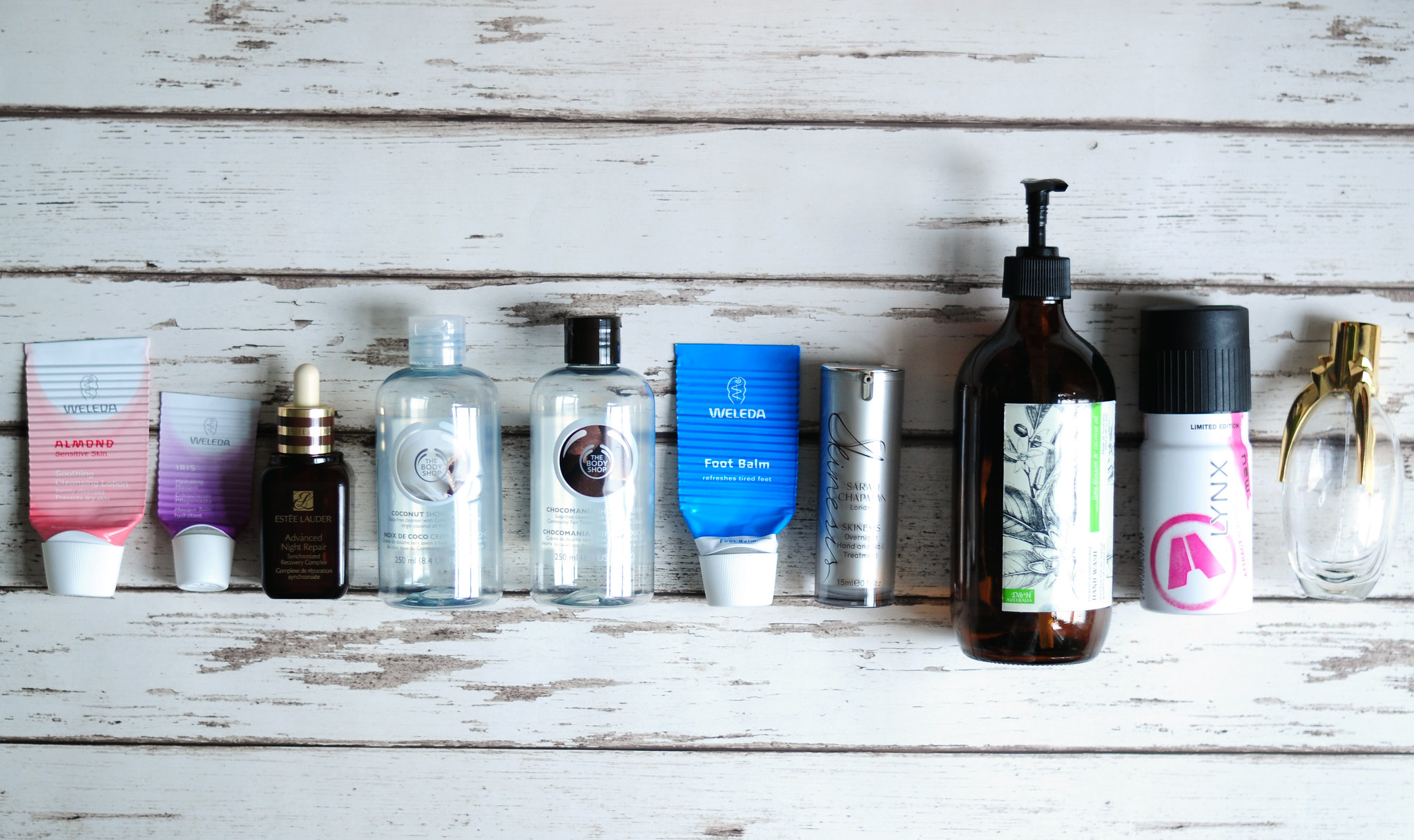This overhead photograph depicts a weathered white-painted wooden deck, its surface roughened and peeling in various areas. At the center of the image, a collection of different skincare and personal care products are arranged. Among them is a tube labeled "Foot Balm", and several bottles resembling containers for shampoo. One prominent dark brown bottle features a push-button dispenser, likely for moisturizer. The assortment includes clear plastic bottles and one item that appears to be deodorant, though much of the text on the products is difficult to discern. The contrasting textures of the aged deck and the modern packaging create a visually intriguing composition.